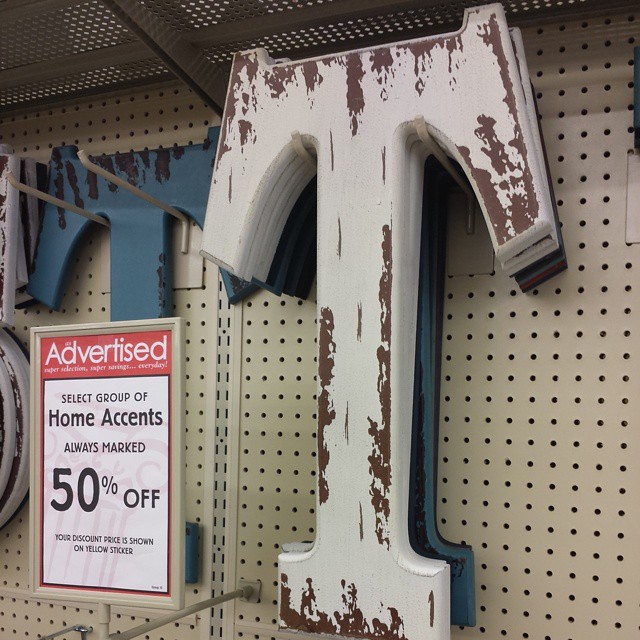This image features a display resembling one from Hobby Lobby, showcasing a variety of home accent items, prominently advertised with a "Select Group of Home Accents Always Marked 50% Off" sign. The discount, clearly indicated by a yellow sticker, is easily visible. Among the displayed items are assorted decorative letters, ideal for various DIY projects. The letters feature diverse designs: one particularly stands out with a distressed look, combining white with brown and rust-colored patches, giving it a weathered, chipped appearance. Another letter has a roughly-hewn texture with a blue hue, enhancing its rustic charm. These items are neatly arranged on pegboard and hooks, characteristic of in-store displays. The overall presentation, marked by a mix of textures and discounted prices, strongly suggests it hails from the home accents section of Hobby Lobby.